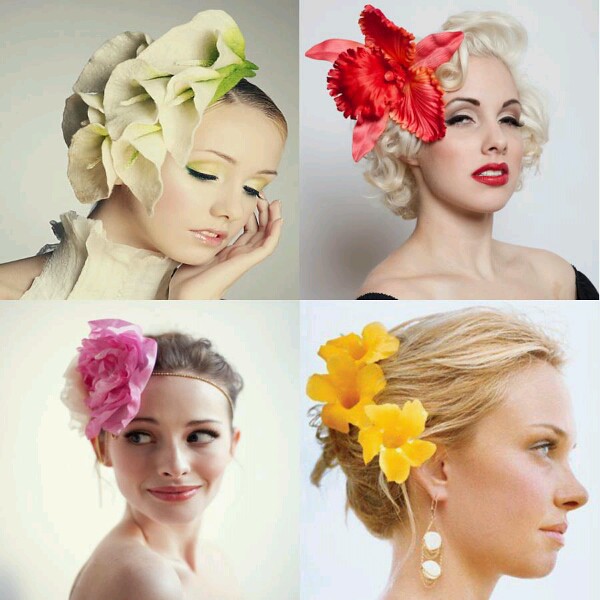This image is a collage of four close-up portraits of white women with variations of blonde hair, set against slightly different soft white or beige backgrounds. Each of the four equal-sized squares within the larger composite photograph features a different woman adorned with elaborate flowers and distinct makeup styles, emphasizing their unique beauty.

In the top left square, a blonde woman gazes downward towards the lower right. She wears a high-neck, shoulderless white blouse and has pale green and yellow eye makeup. Her hair is arranged with a cascade of calla lilies, creating a floral hat-like effect.

The top right square features a platinum blonde woman reminiscent of Marilyn Monroe. Wearing a black off-the-shoulder dress, she sports deep red lipstick and smoky eye makeup. Her hair is styled in soft curls, and a vibrant red orchid is perched just above her right ear.

The bottom left square captures a young woman looking over her right shoulder towards the left of the image. While her attire is not visible, her bare shoulder and narrow headband with a large pink English rose above her right eyebrow define her look.

In the bottom right square, a blonde woman with her hair styled in a chignon gazes to the right. She wears a distinctive drooping earring with two white blocks and has three buttercup orange flowers tucked into her hair.

Each woman's unique floral adornment and distinct makeup highlight their individual styles, coming together to create a unified portrayal of diverse beauty.